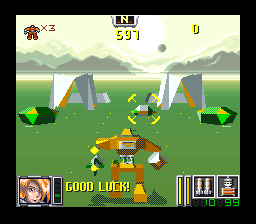In this image, we see a screenshot from an unidentified video game. At the bottom of the screen, the words "Good Luck" are displayed. In the foreground, there is a primitively drawn orange robot-like figure with large shoulders and a relatively smaller head. The background features a green field with two simplistic, silver tent-like structures. Above the horizon, a gray mountain range is depicted, with a stark white sky above it, suggesting a minimalist artistic style.